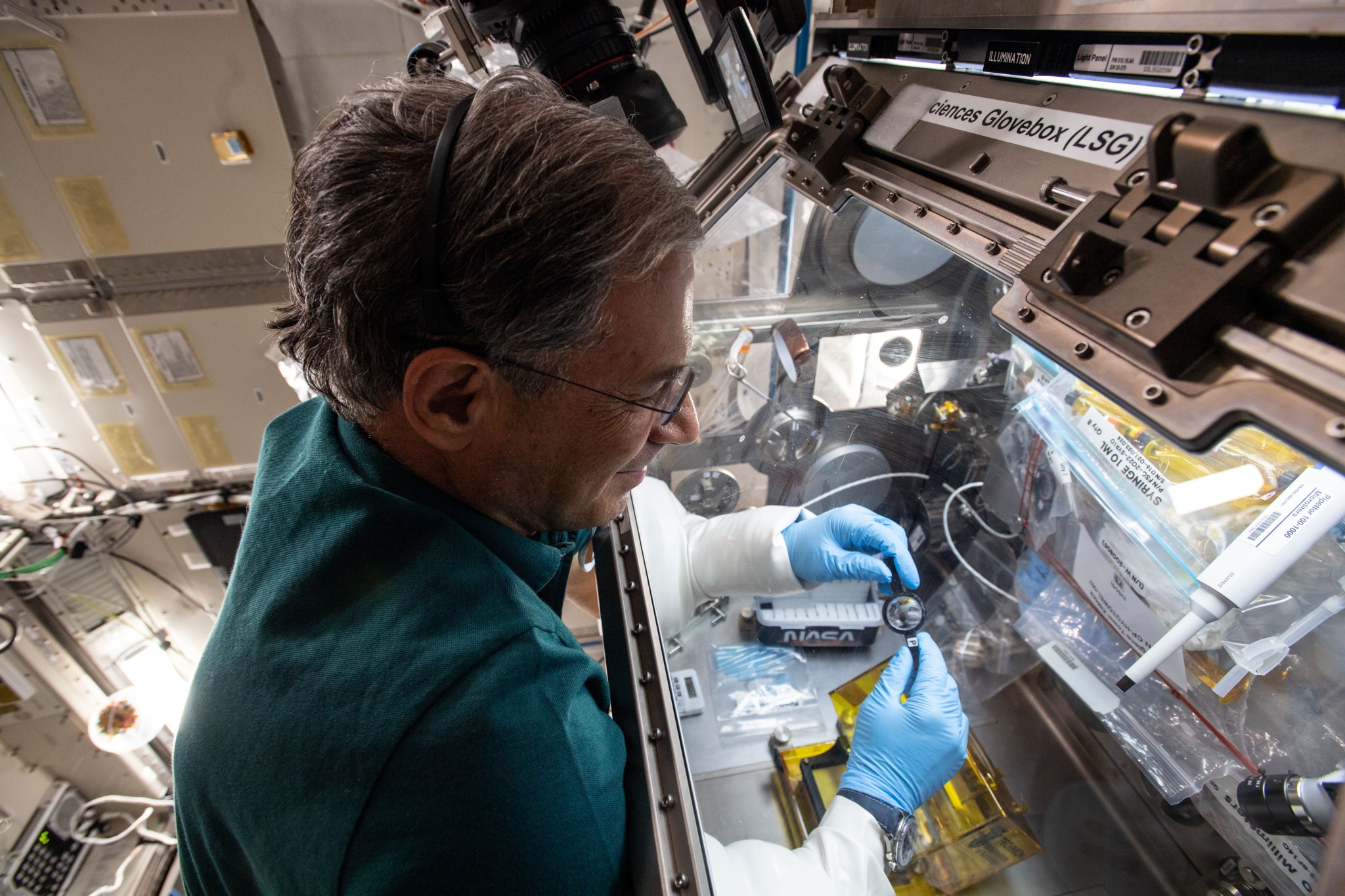A color photograph captures a NASA technician, possibly an astronaut, working meticulously in a high-tech laboratory environment. Dressed in a green shirt and bifocal glasses with graying hair parted to the side, the technician's profile is visible as he engages in a precise task. His hands are inside a specialized containment unit known as a "glove box" (labeled "Glove Box [LSG]" in black text on white), indicating a sterile or controlled environment. He is handling what appears to be a magnifying device, with his hands protected by blue gloves that extend through the box's glassed-in arm ports. The containment unit itself is constructed of silver metal with large hinges, and it features other devices including a yellow box, a white rod resembling a telescope, and a box bearing the NASA insignia. The backdrop is a wall adorned with various pieces of electronic machinery, wires, and buttons, suggesting a complex and advanced setting for scientific or aerospace research.